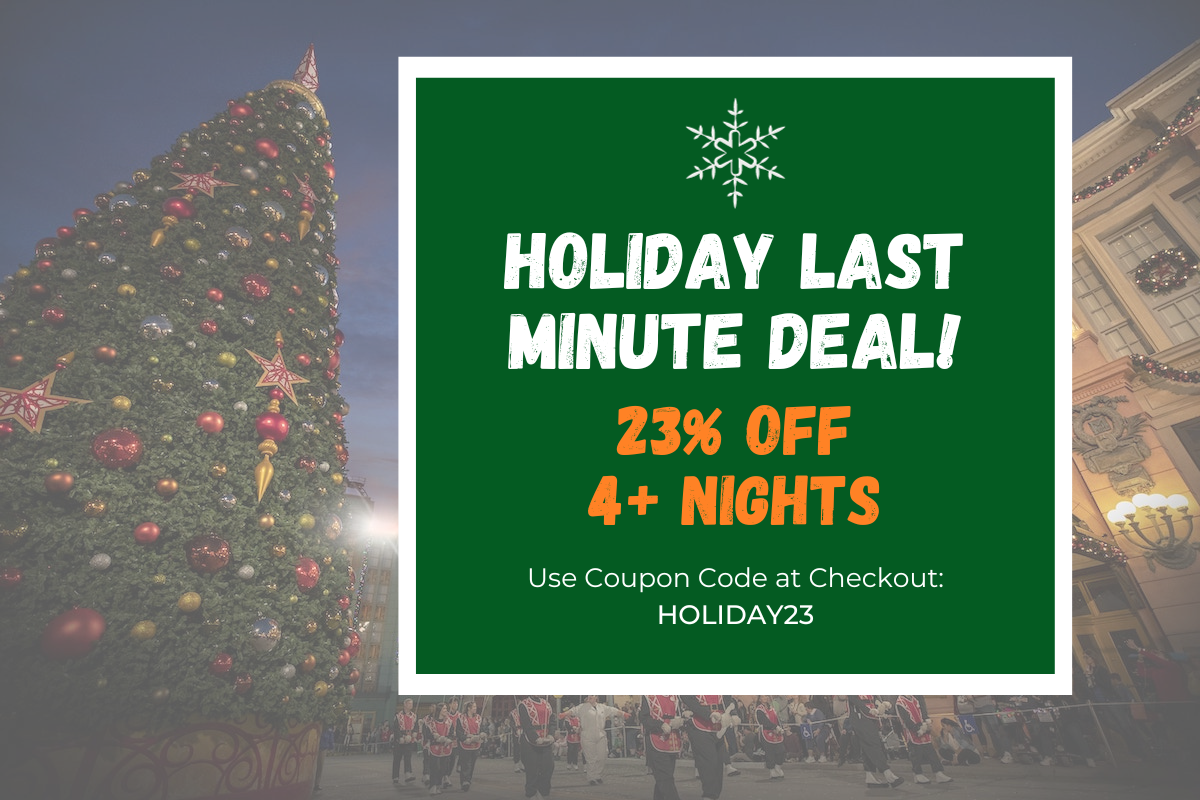Screenshot of a holiday-themed advertisement on a website featuring a last-minute deal. The ad prominently displays a green field with the text "HOLIDAY LAST MINUTE DEAL" written in a hand-drawn capital letters style, along with a white snowflake graphic at the top. Below this in bright orange, the text reads "23% OFF" followed by "4+ NIGHTS." The instructions "Use coupon code at checkout" appear in a standard font, with the coupon code "HOLIDAY23" highlighted in bold capital letters.

The advertisement is positioned slightly to the right of the center of the page. Behind the ad is a photograph with a semi-transparent white overlay depicting an outdoor holiday parade. The scene features a large, fully decorated public Christmas tree and a series of neoclassical buildings in the background. In the parade, band members dressed in red tops and black pants play various instruments, although specific details are hard to discern. A man dressed in white with his arms extended leads the band. On one side of the street, a roped-off area holds onlookers who are watching the festive display. The surrounding buildings are adorned with wreaths, garlands, and multiple Christmas decorations, featuring a stone facade with sections in yellow and cream colors.